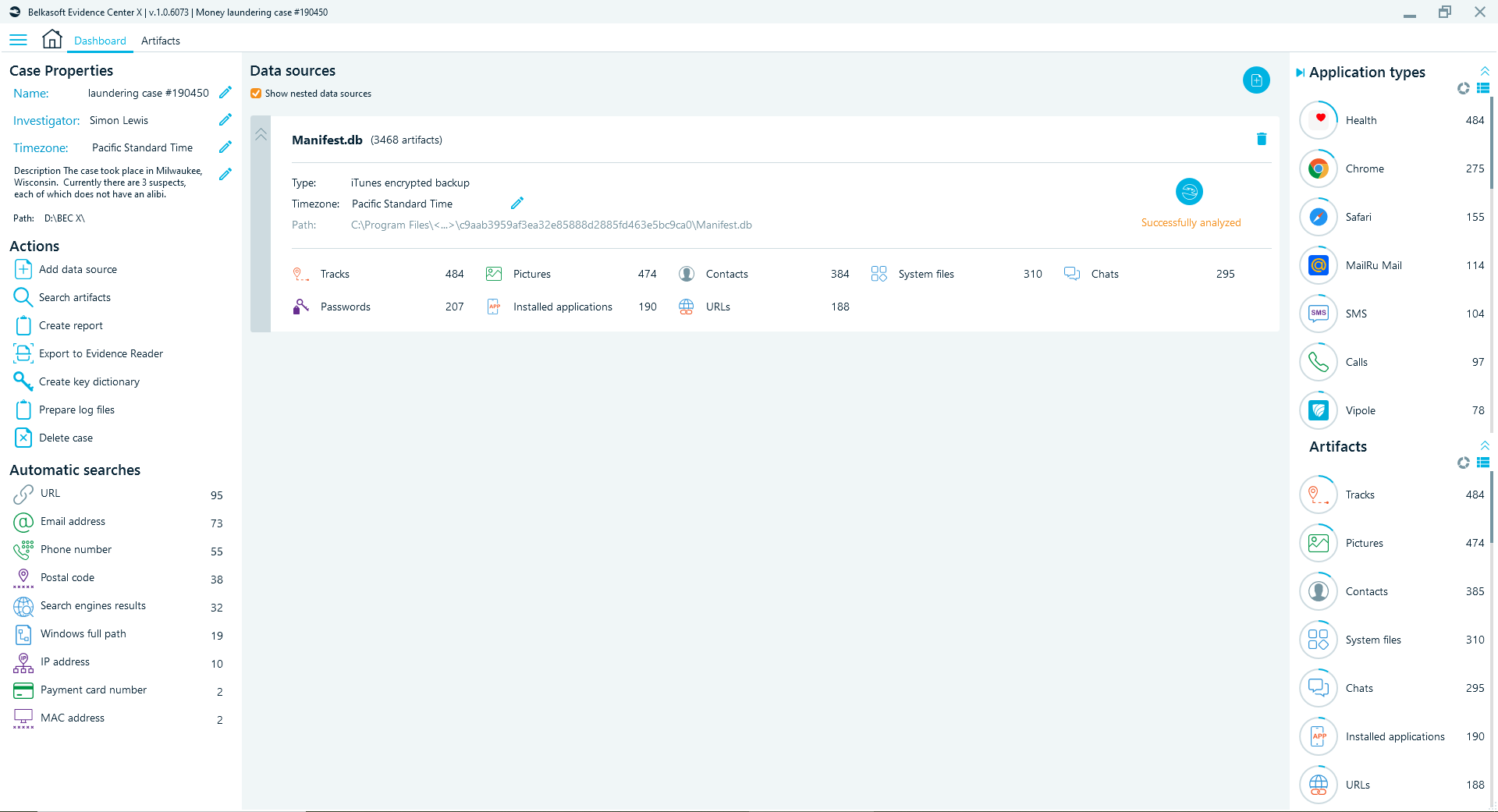This is a detailed screenshot of a website used for digital investigations, specifically the Belkasoft Evidence Center X, version 1.0.6073. The case displayed is labeled as "Money Laundering Case 190450."

In the top left corner, the interface highlights key case properties:
- **Case Name:** Laundering Case
- **Investigator:** Simon Lewis
- **Time Zone:** Pacific Standard Time

A brief description notes that the case occurred in Milwaukee, Wisconsin, and currently involves three suspects, each of whom lacks an alibi. Additionally, the path to the case file on the investigator's computer is specified, although it is not visible in the screenshot.

Further down on the left side, there are actionable options including:
- Add a data source
- Search artifacts
- Create a report

The central pane of the interface lists data sources, with an example being "Manifest.DB," which contains 3,468 artifacts. This suggests the software is utilized by investigators to systematically organize and manage complex cases, facilitating easier access to and analysis of critical information.